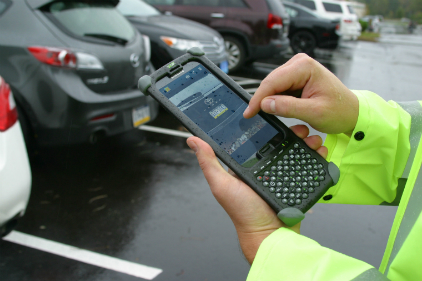In a rain-soaked parking lot, a figure—likely a parking attendant or meter maid—stands by the back corner of a white car, dressed in a high-visibility yellow raincoat. The wet asphalt glistens beneath a gentle drizzle, reflecting the overcast sky. The attendant's left hand holds a small handheld device resembling a tablet or an older model of a phone with keys at the bottom. Their right hand appears to be typing or pointing at something on the device's screen. Around them, blurred slightly by the rain, are six parked cars, including a white, gray, black, and brown car. The attendant might be checking the license plates, possibly verifying parking fees, as marked by the presence of various car license plates in the background.